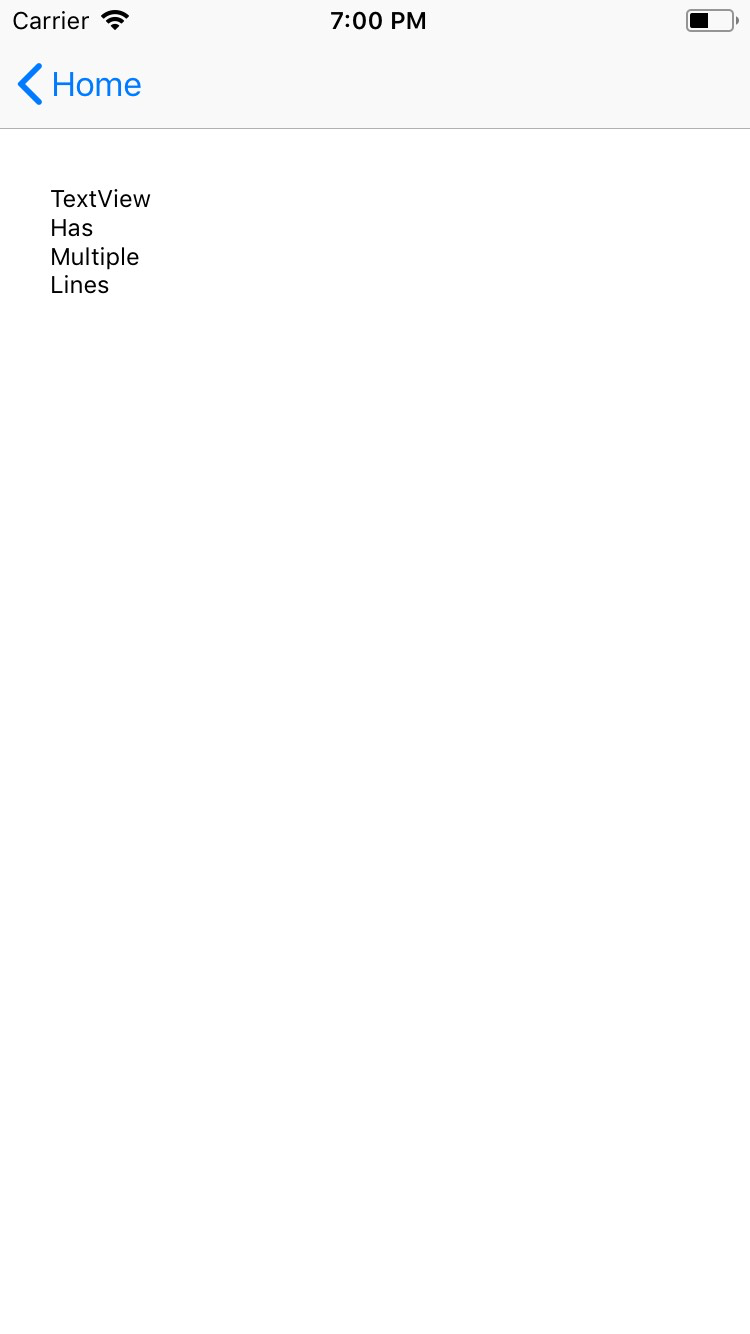**Screenshot of Text View App Functionality**

This screenshot demonstrates the Text View app on a smartphone. 

In the status bar at the top of the screen, the left corner displays "carrier," a placeholder typically indicating service providers such as Verizon or AT&T. Adjacent to this, there's a Wi-Fi signal icon, and centrally positioned is the time, "7:00 PM." The rightmost side features a battery icon.

Below the status bar, a gray navigation bar is visible, with the word "Home" in blue lettering accompanied by a left-pointing arrow, suggesting a back navigation option.

The main portion of the screen is predominantly white, displaying black text in several lines. The text reads as follows:

- "text view"
- "has"
- "multiple"
- "lines"

This indicates the app's capability to accommodate multiple lines of text. The purpose of this screenshot is to illustrate the app's functionality, specifically how users can either write in a multiline format or compose extended paragraphs within the application. The clean and minimalistic design aids in showcasing the app's usability for various writing needs.